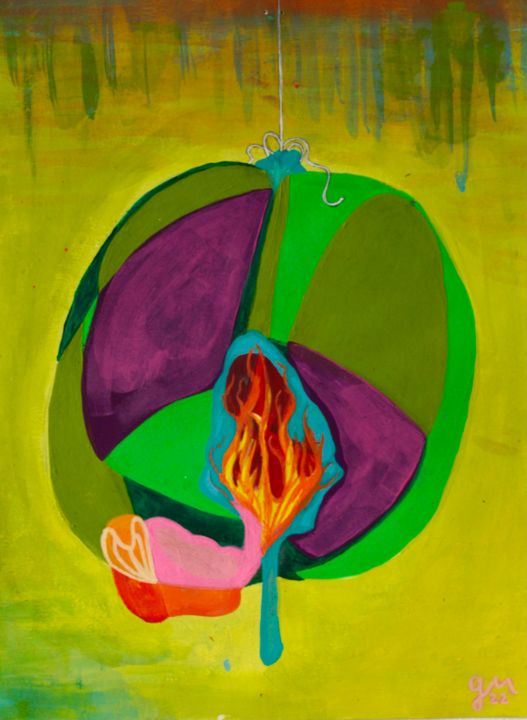The image features an abstract art piece, created with a vivid assortment of paints, centered around a circular configuration filled with distinct patches of colors. This central circular shape incorporates a variety of greens—bright green, darker green, and forest green—interwoven with bright purples. Near the bottom middle of this shape, a tree or leaf-like outline emerges, painted in blue and teal blue hues. At the center of this outline, vibrant splotches of red, orange, and yellow evoke the appearance of flames, suggesting a dynamic interplay of elements.

Adjacent to this fiery motif and positioned toward the bottom left within the circle, there's an abstract form composed of pink, red, orange, and yellow tones, which might suggest anatomical references, like human organs. This entire circular shape appears to be suspended from the top of the image by a white string-like element, subtly connecting it to the upper section of the painting.

The background amplifies the central theme with a blend of bright, almost acidic green and darker green splotches, punctuated by occasional additions of red, blue, and further green hues near the top. The overall effect is a harmonious yet complex interplay of colors and abstract forms. The painting is signed in light pink located in the bottom right-hand corner, adding a personal touch from the artist.